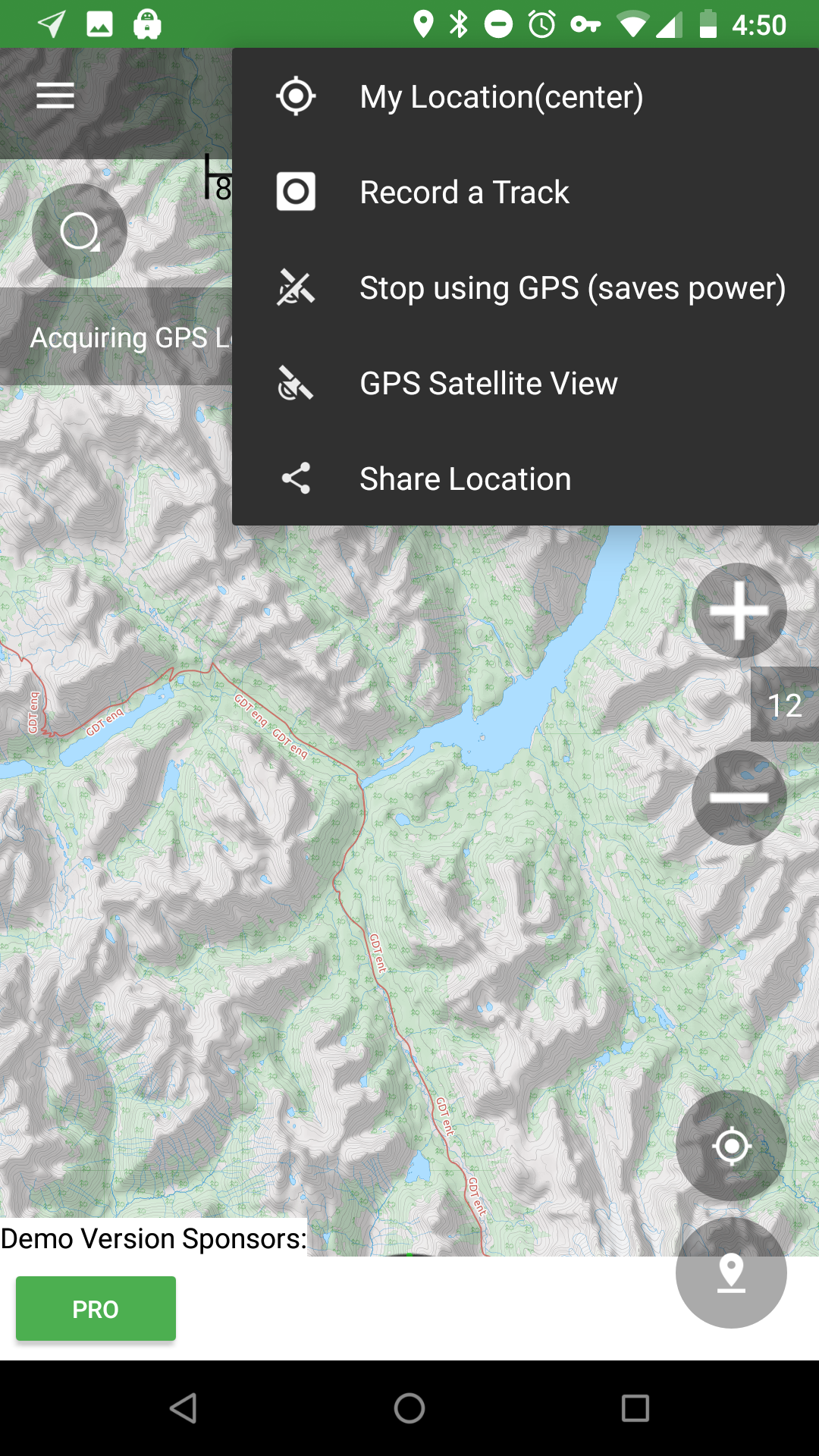This screenshot depicts an image of a map interface. At the top, against a green header, a series of white icons are displayed: a pin, Bluetooth on, an alarm clock, a key, Wi-Fi, signal reception, battery status, and the current time (4:50). On the right side of the green header are these icons. Over the map, a black box with white text is open. The text in the box, listed from top to bottom, includes: "My Location Center," "Record a Track," "Stop Using GPS" (with a note about saving power), "GPS," "Satellite View," and "Share Location." The map itself is predominantly light green, showcasing tan and brown areas that suggest mountainous and rocky terrains. Beneath the map, the background is white, and there is a green action button on the left labeled "PRO." Just above this button, in small black text, it reads "Demo Version Sponsors."